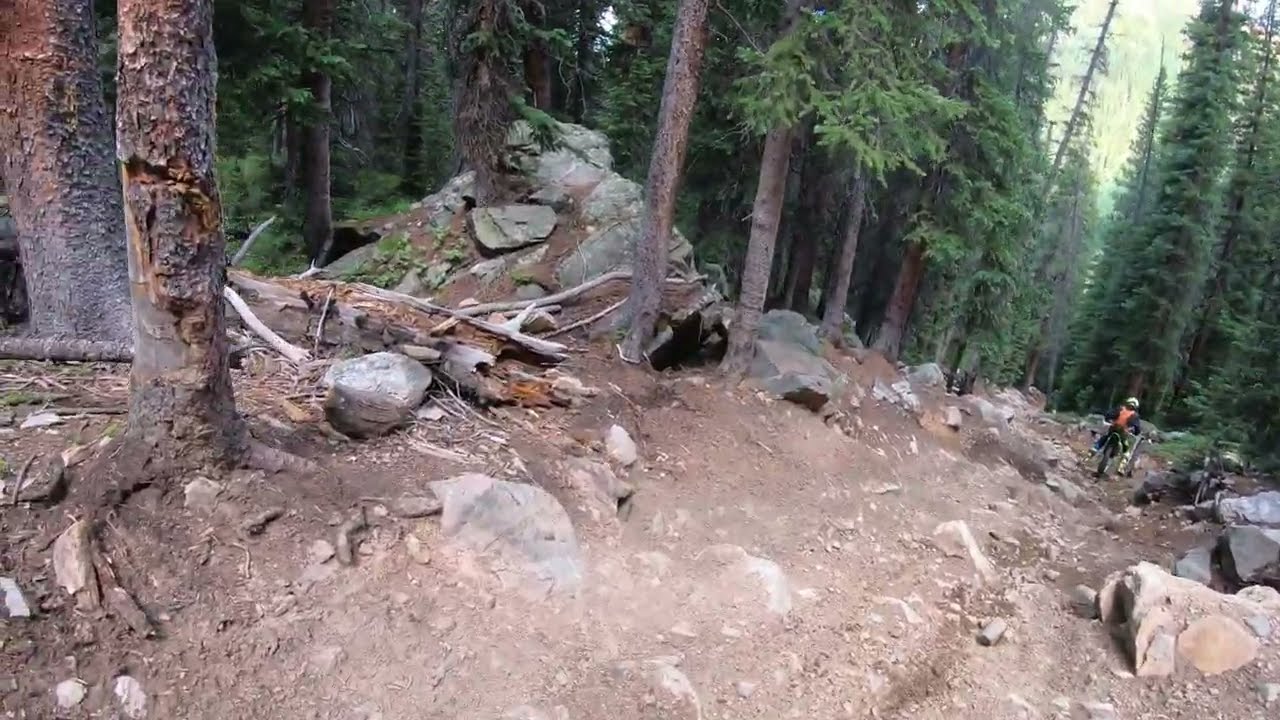The photograph captures a rugged, mountainous terrain with a person navigating a rocky, unmarked path on a mountain bike. The individual is wearing a helmet and an orange reflective vest over a black jacket. The path, which appears to be more of a rough trail forged through the wilderness, is littered with dirt, various sized rocks, and sizable boulders, indicating a challenging ride. Tall pine trees dominate both sides of the scene, with some showing signs of decay, and fallen, rotting logs accentuating the wild, untamed nature of the setting. In the background and stretching into the distance, a dense forest of towering trees can be seen, while the sky above is filled with a mix of clouds, casting a muted light over the landscape. The path curves to the right, leading the eye toward the biker who is skillfully maneuvering through this rugged, scenic environment.